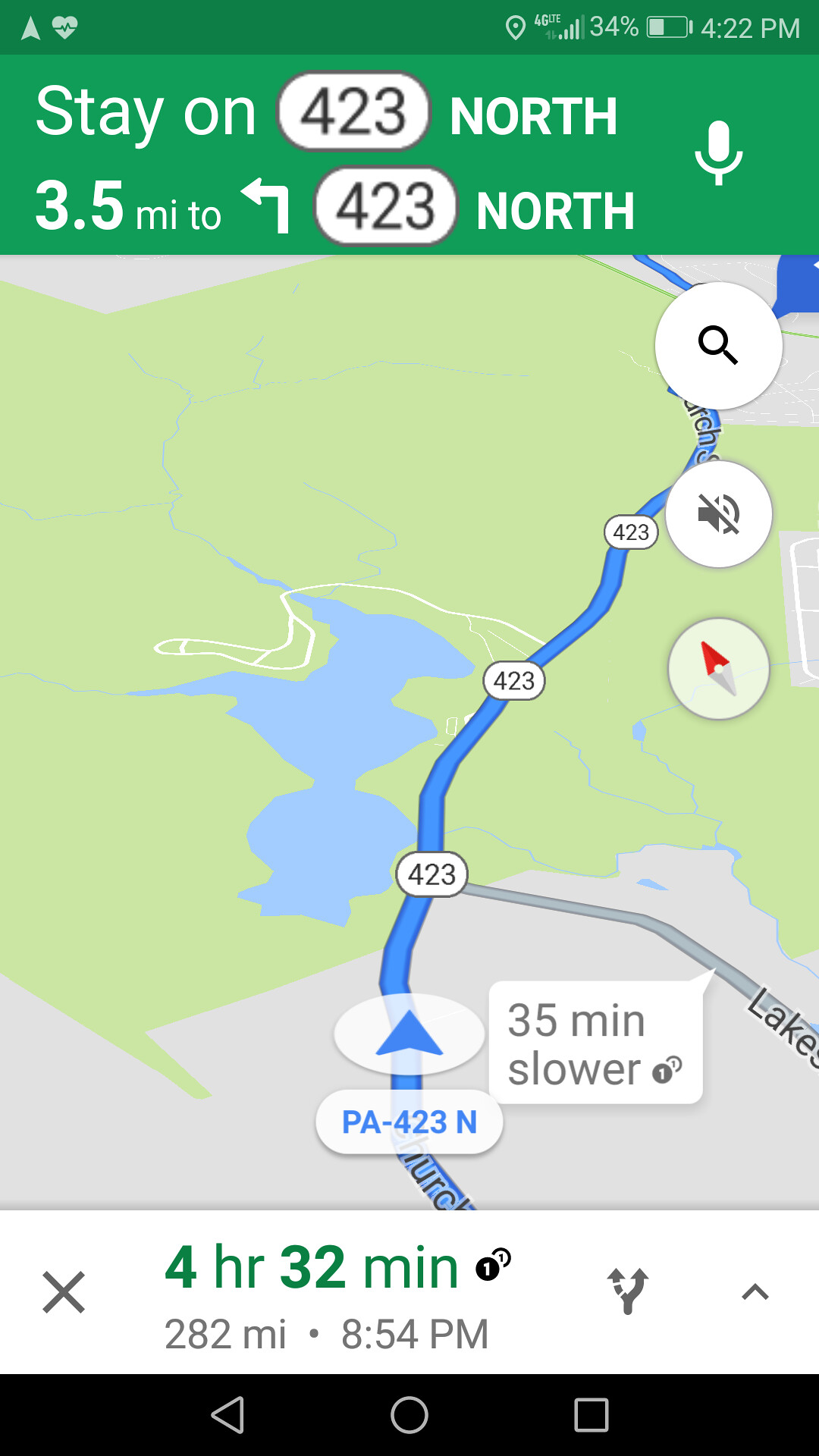A screenshot captures a smartphone displaying a navigation map. The device indicates it has 34% battery life remaining, and the current time is 4:22 PM. The map, prominently featured, guides the user to stay on Route 4.23 North for 3.5 miles before making a left turn, with this instruction highlighted in green text at the top. A microphone icon is also visible, suggesting voice command functionality. The map shows a green area with a blue section at the bottom. A blue line traces a route from the top right to the bottom middle of the map, marked with the number "4.23." The route information includes a note stating "35 minutes slower" at the bottom of the line. The lower part of the screen features a white banner with a green background, displaying the estimated travel time as 4 hours and 32 minutes, covering a distance of 382 miles, with an expected arrival time of 8:54 PM.